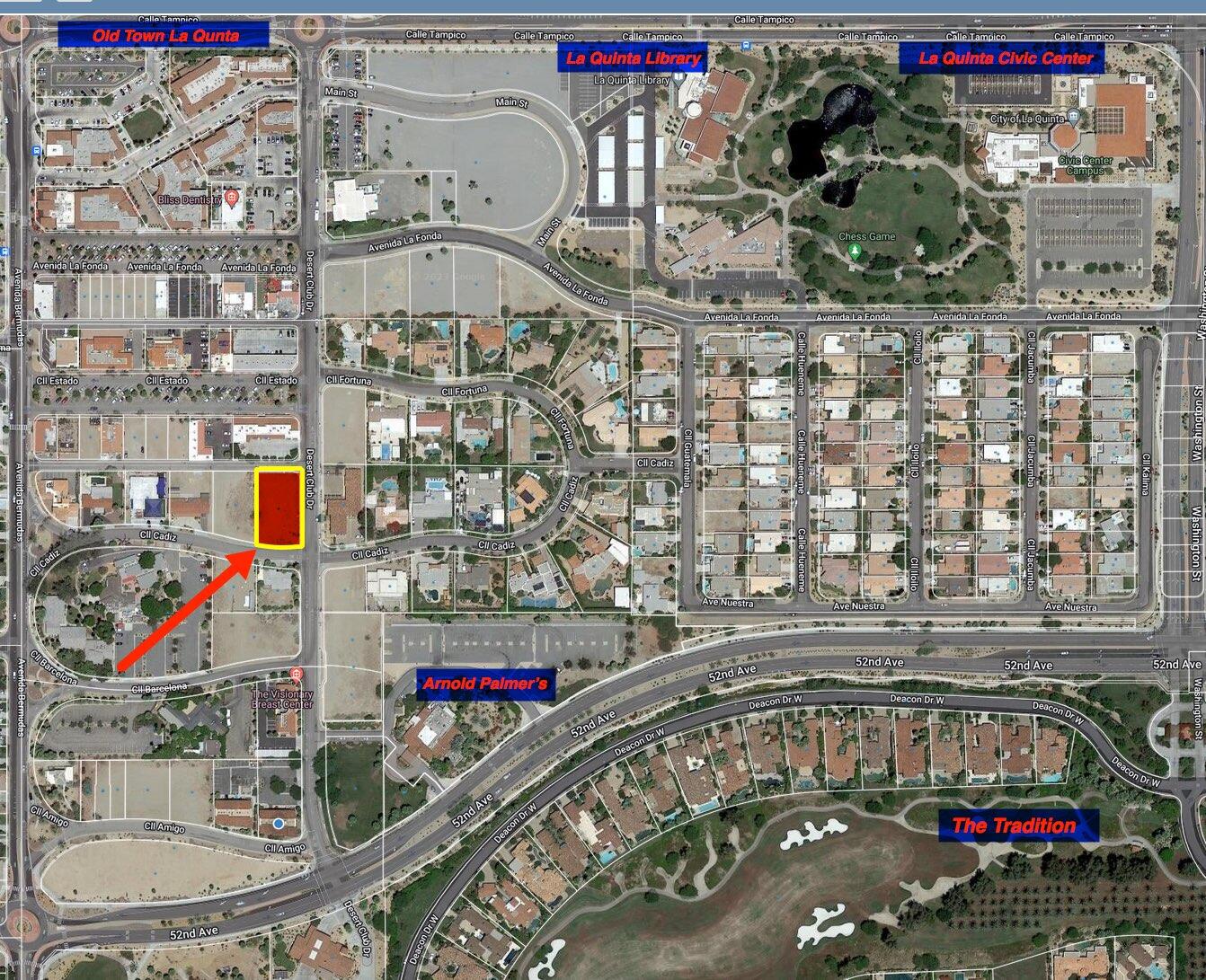This image is a detailed satellite map of a city area, showcasing buildings, streets, and blocks. The image prominently features a specific rectangular area, colored in red with a yellow border and highlighted by a red arrow, located about halfway down on the left side. There are several points of interest labeled with blue banners and red text, including "Old Town La Quinta" in the upper left, "La Quinta Library" centrally, and "La Quinta Civic Center" in the upper right. Towards the bottom, notable labels include "Arnold Palmer’s" next to a building with a large empty parking lot and "The Tradition" by the golf course. The image depicts a vibrant urban landscape with tree-lined streets and various detailed annotations of street names such as 52nd Ave, Deacon Drive West, Circle Cadiz, Avenida La Fonda, Main Street, and Cal Tampico. Additionally, the map shows a neighborhood with many houses, a park in the upper right, and a double-lane highway curving past another neighborhood adjacent to a golf course.